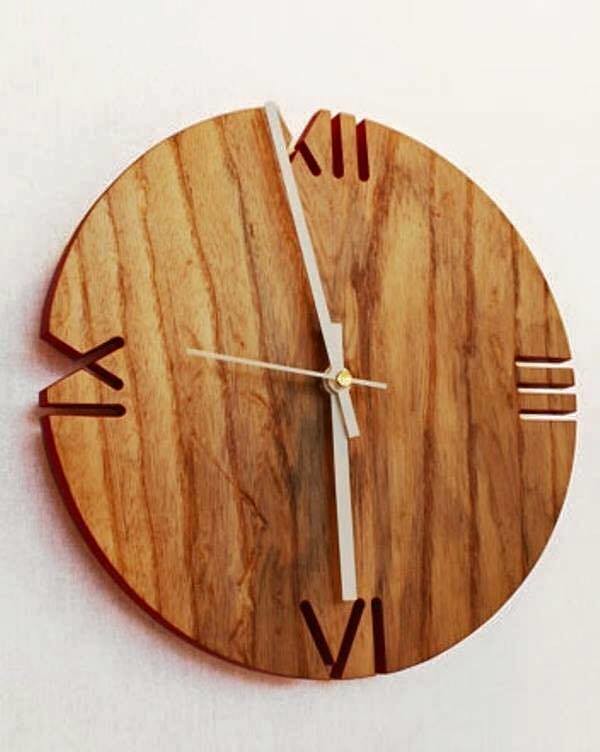A wooden clock features intricately carved Roman numerals against a green background. The right hand points to VI, the left hand to XII, and a second hand hovers between XI and IX. Both the III and XII numerals are meticulously cut out of the wood, adding depth and texture to the design. The clock face is adorned with brown circles and intersected by dark, scrunched lines, enhancing its rustic, handcrafted aesthetic.